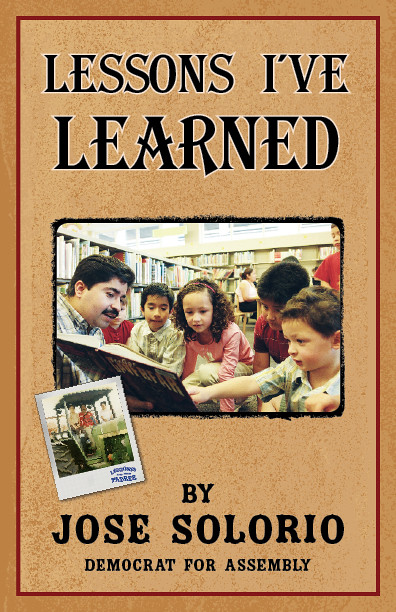This political poster features a brown background with a darker brown-red border. At the top, bold black letters proclaim "Lessons I've Learned." The bottom of the poster attributes the source with the text "by Jose Solorio" and specifies his candidacy with "Democrat for Assembly" in smaller black letters.

The central image depicts Jose Solorio engaging with a group of five or six children, pointing at a book in what appears to be a library, evidenced by the shelves of books in the background. Solorio appears to be presenting educational material to the students, illustrating his commitment to education.

Below this primary image, a smaller, postage stamp-sized picture shows a figure beneath a canvas tent, presumably Solorio, delivering a speech. This visual element reinforces his active political engagement and dedication to public service.